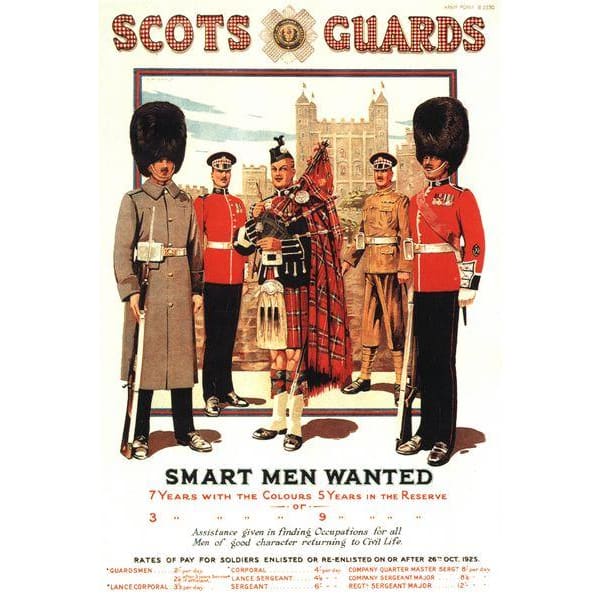This image is a scan of an old recruitment poster for the Scots Guards. At the top of the poster, the title "Scots Guards" is prominently displayed in checkered red and white lettering. The poster features a vibrant hand-drawn illustration of five men, each showcasing various uniforms associated with the Scots Guards. 

From left to right, the figures include a soldier in a long beige coat with a belt and a rifle resting on the ground, wearing a tall fur hat. Next to him stands a soldier in a red uniform with black pants and the iconic tall black fur hat commonly seen during the changing of the guard at Buckingham Palace. Another figure is adorned in traditional Scottish attire, including a red plaid kilt, black hat, and is playing the bagpipes. Additional figures include a soldier in a tan uniform with a black brimmed hat and another in a typical red jacket and black pants ensemble.

The text below the illustration reads, "Smart Men Wanted. Seven Years with the Colours, Five Years in the Reserve," followed by information about the rates of pay, ranging from guardsmen to various levels of sergeant. The rates of pay are specified as follows: guardsman at $2 per day, lance corporal at $2.30 per day, corporal at $4 per day, lance sergeant at $4.50 per day, sergeant at $6 per day, company quartermaster sergeant at $8 per day, company sergeant major at $8 per day, and regiment sergeant major at $12 per day. Additional assistance is offered in finding occupations for all men of good character returning to civil life. The poster also notes that the rates apply to soldiers enlisted or re-enlisted on or after 26 October 1925.